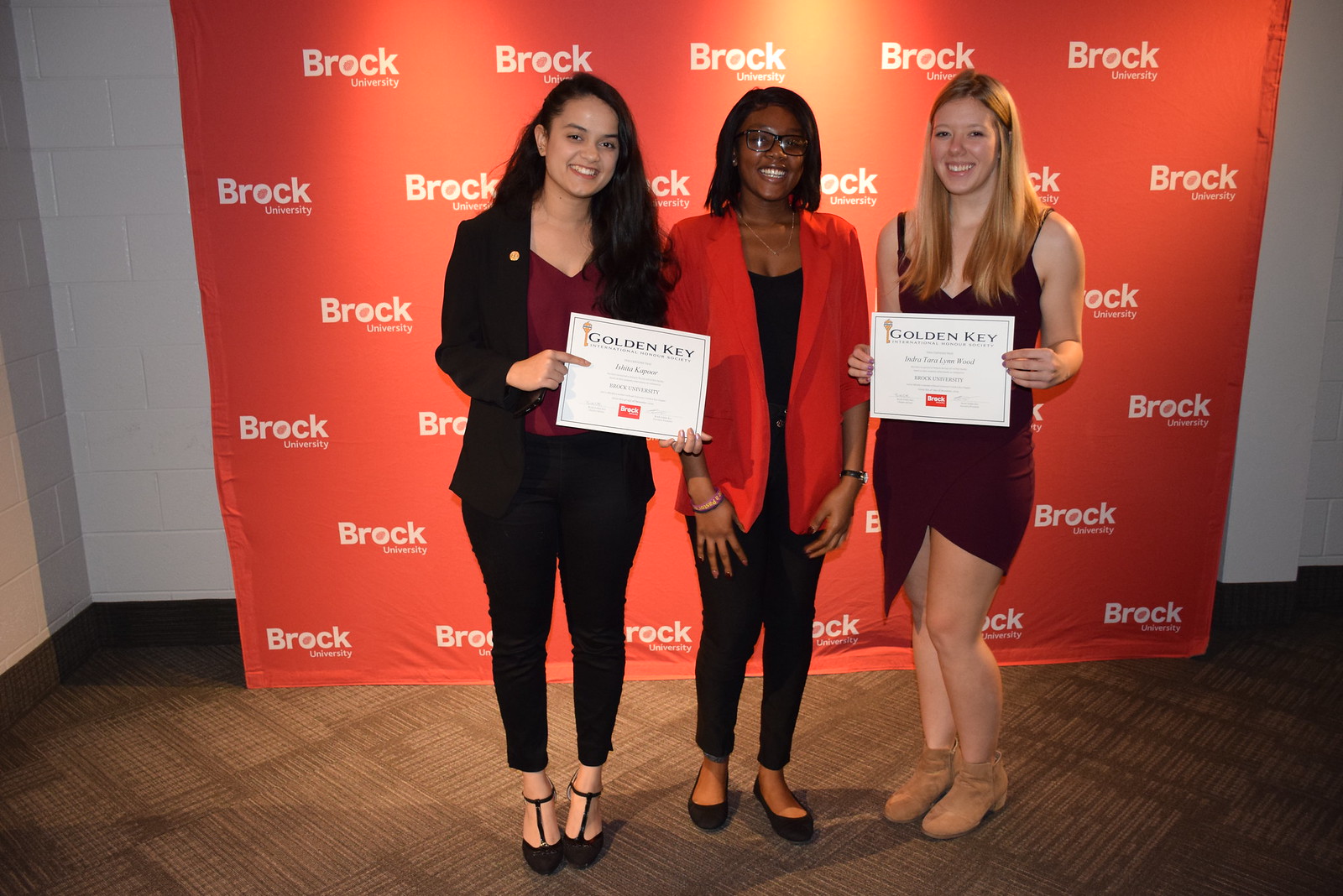The color photograph captures three professionally dressed women standing in front of a red backdrop with white repeating text that reads "Brock University." Behind the backdrop is a white painted cinder block wall. The women are posed in front of the backdrop on a light gray floor.

From left to right, the first woman has long dark hair and is dressed in a black blazer, black pants, and a burgundy top. She is holding a white certificate that reads "Golden Key." The second woman in the center, with a black bob haircut and glasses, is wearing a red cardigan over a black top with black pants and black ballet flats. The woman on the right has long blonde hair and is dressed in a strappy burgundy dress that comes to mid-thigh with tan ankle boots, also holding a white certificate labeled "Golden Key."

The women are beaming with joy, and their formal attire enhances the celebratory and professional atmosphere of the scene.